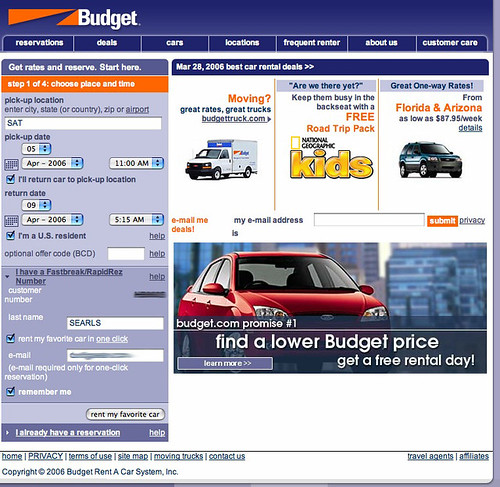This is the Budget.com website. In the upper left-hand corner, there's an elongated, slanted, orange triangle pointing towards the upper right. Below it, there's a smaller, upside-down orange triangle, with its right side aligned with the letter 'B' in the logo. The logo itself features the word "Budget" in a somewhat bulky, white font with a capital 'B' followed by lowercase letters and a period at the end.

Below the logo, there's a navigational menu with a white background and rounded edges. The items in the menu are separated by white lines and listed in small, bold, white font. The items are: Reservations, Deals, Cars, Locations, Frequent Renter, About Us, and Customer Care.

The main background of the website is white, transitioning into a rectangular menu with rounded corners towards the left. The top section of this menu has a dull navy blue strip with white lettering that reads "Get Rates and Reserve. Start Here." Below this, there's a thin white line separating it from a bright orange banner with white font that says "Step 1 of 4: Choose Place and Time."

The next section of the menu has a bluish-light-gray background. In dark blue, bold font, it says "Pick-Up Location." Below this, in a dark blue, non-bold, slightly smaller font, it reads "Enter city, state (or country), zip, or airport," with "airport" underlined, likely indicating that it is clickable.